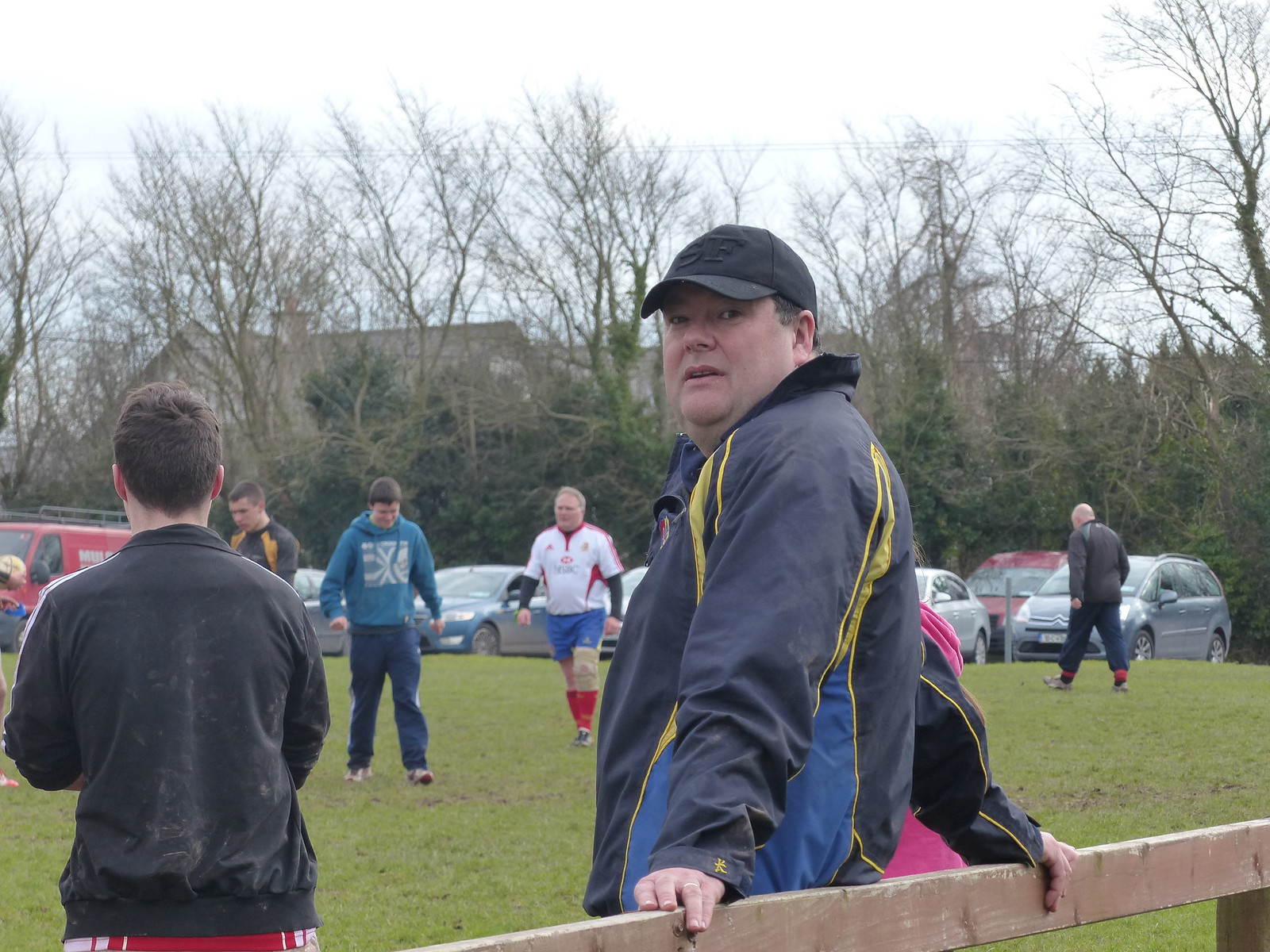In this outdoor daytime photograph, an older, larger man leans on a weathered wooden fence, painted brown but worn to a gray in many spots. He wears a black baseball cap embroidered with "SF" and a blue windbreaker with yellow stripes and lighter blue side panels. The man, whose face shows a surprised expression, faces the camera while his body is oriented toward a sprawling green field, where multiple people—many in sports-type clothing and hoodies—move about. In the background, across the field, a parking lot is visible, lined with numerous vehicles. The day appears overcast, with a sky transitioning from blue to bright white. Near the man, to his left, stands a young boy in a dusty black coat over a red jersey, and to his right, someone in a pink coat. Further back, additional individuals, including an older man in a white jersey with red accents and another in a dark windbreaker and tennis shoes, populate the scene. The distant horizon features a mix of barren trees and a few pine trees.